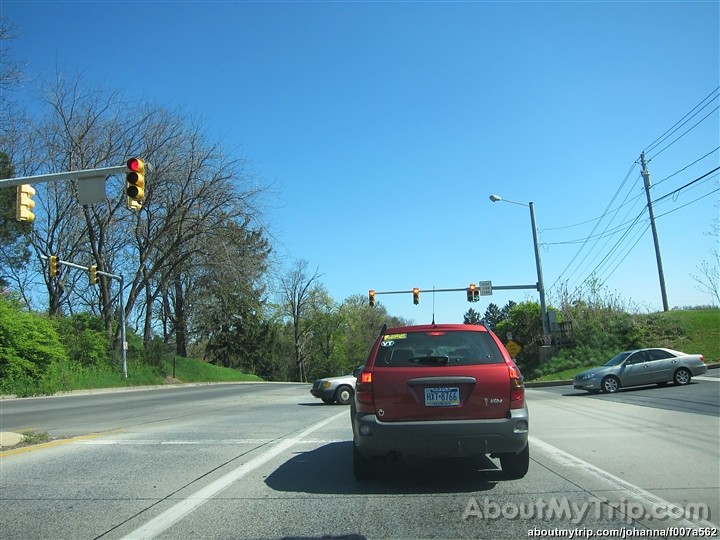This photograph, presumably taken from a dashcam inside a moving car, captures a daytime scene at an intersection. In the foreground, a red SUV with a gray bumper and two stickers on the top left corner of its back windshield—one yellow, one white—is stopped at a red traffic light. The traffic light is mounted on a large, gray, horizontal pole to the left and displays a red light in yellow housing. The road, light gray with visible wear and cracks, features white stripes delineating the lanes. A silver car is crossing the intersection from left to right, followed by a white car whose front end is just visible adjacent to the red SUV. The sky is a vibrant blue with wisps of white clouds.

The image also reveals a landscape of leafless trees on the left with additional trees and bushes bearing dark green foliage in the distance. Grass and bushes in varying shades of green line both sides of the road near the intersection. On the right side of the image, across the intersection, more greenery and a yellow sign are visible. The photograph includes a watermark on the bottom right, displaying "aboutmytrip.com" in opaque white text, along with "aboutmytrip.com/johanna/F007A5672" in smaller white text.